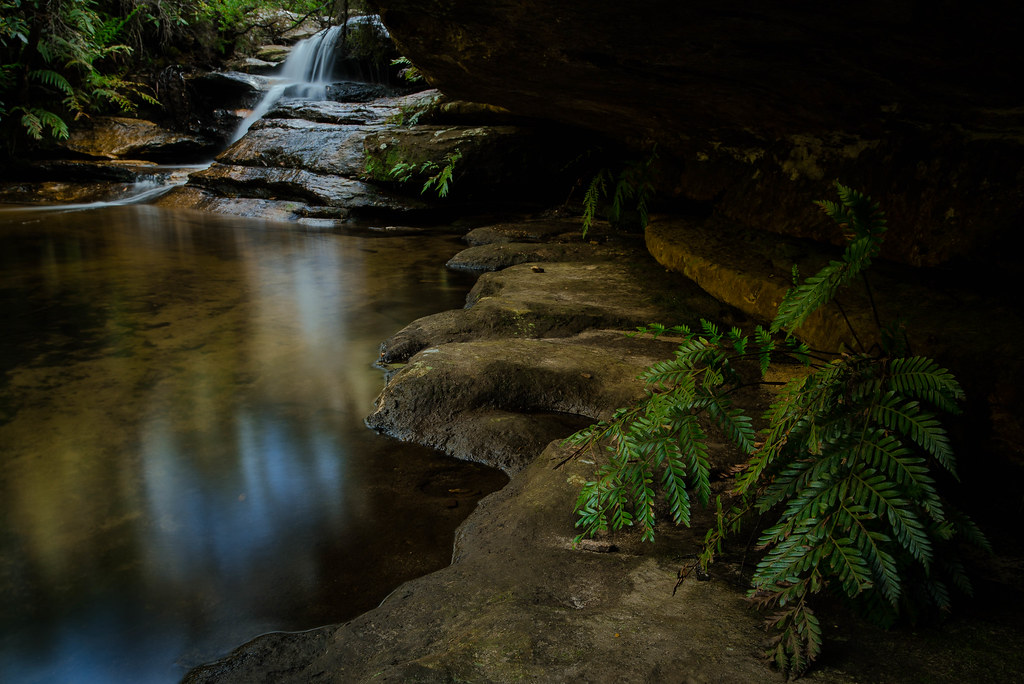The AI-generated image showcases a serene, rocky shoreline at the base of a small waterfall situated towards the top left. The waterfall cascades down several rocky tiers, eventually feeding into a shallow, lazy river or small pond below. The water, predominantly brown and murky, reflects its surroundings smoothly, devoid of any ripples. Green vines and shrubs sprout from cracks in the grey, moss-covered rocks on both sides. The lush, large leaves of nearby trees add to the scene's verdant atmosphere, while a subtle reflection of the sky is visible on the water's surface. Despite the image's overall dark tone, the detailed landscape evokes a tranquil and natural ambiance.